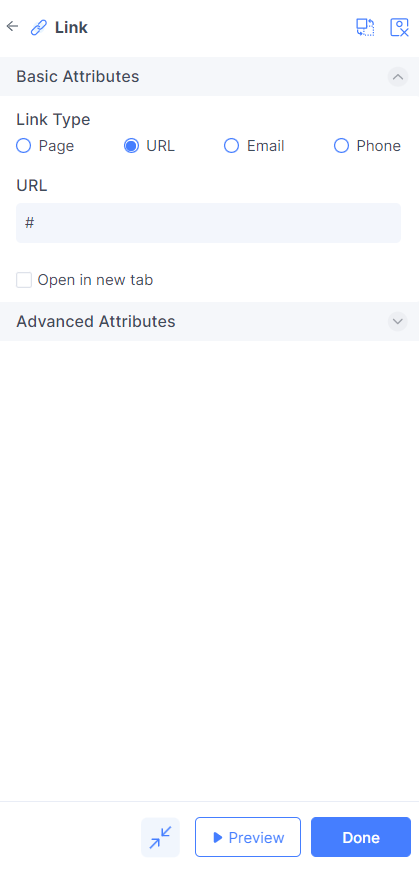The image is a screenshot of a webpage set against a white background. In the upper left corner, from left to right, there is a small gray arrow pointing left, followed by a blue pin icon, and then the word "Link." The upper right corner contains two blurry and indistinguishable icons. Below the header, a light blue banner with dark blue text reads "Basic Attributes," with an upward-pointing arrow at the end of the banner.

Directly underneath this banner, against the same white background, is the section titled "Link Type." This section includes four options, each accompanied by a small circular radio button to the left. The options are: "Page," "URL" (which is selected and filled in), "Email," and "Phone." Following these options, there is a text field labeled "URL" with a blue form line below it for user input.

At the bottom of the screenshot, there is a section labeled "Advanced Attributes." The footer area of the screenshot features two action buttons: one is a white button outlined in blue labeled "Preview," and the other is a blue button with white text labeled "Done."